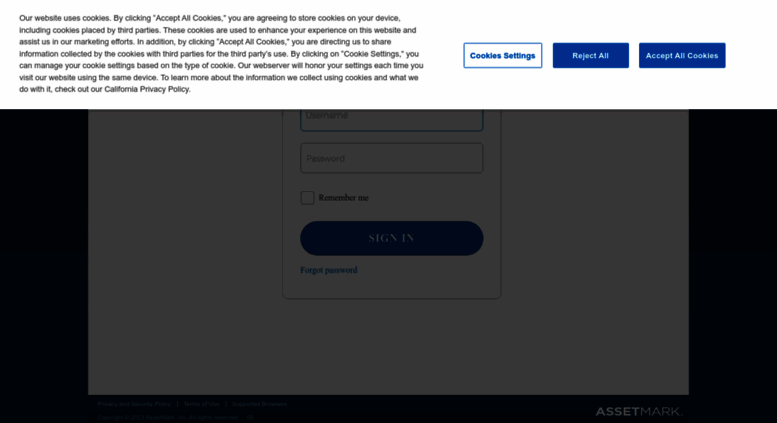The image features a detailed login interface with a privacy notification overlay. At the top left corner, there is a large, semi-transparent text block informing users about cookie usage. The text reads: "Our website uses cookies. By clicking 'Accept All Cookies', you agree to store cookies on your device, including cookies placed by third parties. These cookies enhance your website experience and assist in our marketing efforts. Additionally, by clicking 'Accept All Cookies', you permit us to share information collected by the cookies with third parties for their use. By clicking on 'Cookie Settings', you can manage your cookie preferences. Our web server will audit your settings each time you visit our website using the same device. To learn more about the information we collect using cookies, please visit our documentation and cookie policy pages."

The background is grayed out, emphasizing the login section. The login interface includes fields for "Username" and "Password", alongside the options "Remember Me" and "Forgot Password". The "Sign In" button is a prominent blue oval. The login section is encased in a large white square that contrasts with the dark blue edges framing the entire interface.

Below the login fields, there are links to the "Privacy and Security Policy" and "Terms of Use". Additionally, there is a copyright notice reading, "© 2003 AssetMark, Incorporated, All Rights Reserved." To the far right, the company name "AssetMark" is displayed prominently.

The notification overlay includes options for "Cookie Settings" and "Reject All" in blue and dark blue, respectively, allowing users to manage or decline cookies.